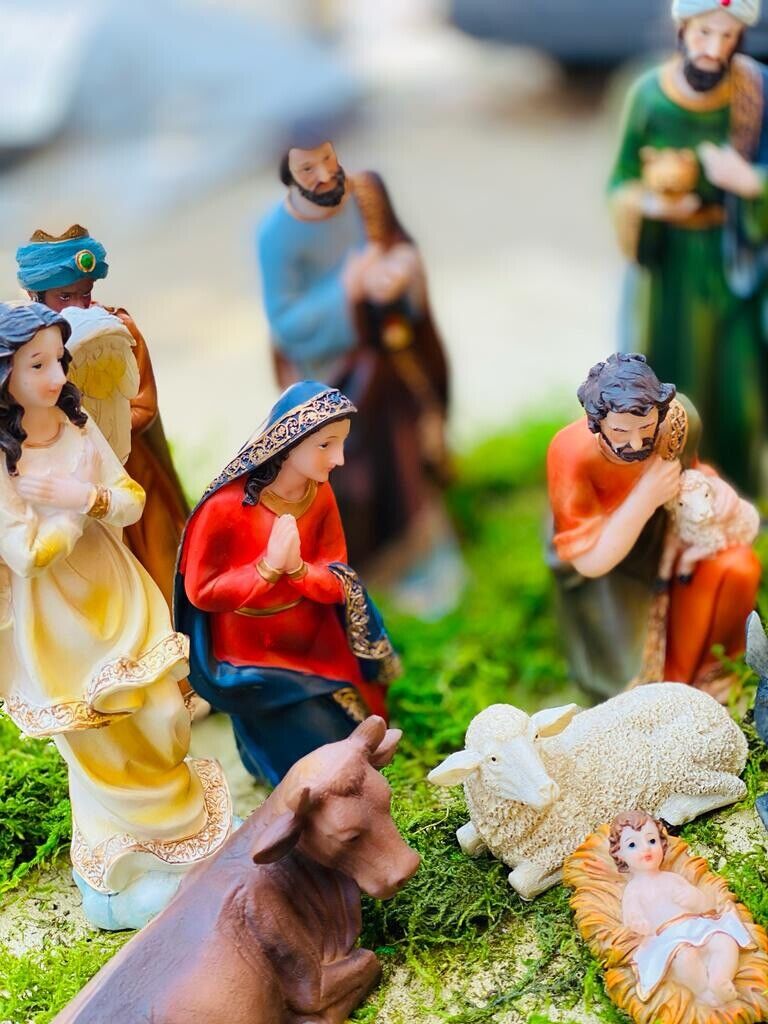This photograph depicts a detailed nativity scene with miniature figurines representing the traditional story of the birth of Jesus. At the center, baby Jesus lies in a small hay-filled manger, surrounded by a brown cow and a white sheep. In the foreground, there is a man holding a lamb on his knee and a woman dressed in a red gown with a blue cape, her hands joined in prayer. Beside her stands another woman in a blue dress with her hands crossed over her chest. Behind her, a figure in a white and yellow robe with angelic wings partially obscures a man donning a blue turban. Further in the background, barely in focus, are a man in a blue shirt with a brown cape and another man wearing a white turban and a green robe, both slightly blurred. The scene is carefully set on patches of vibrant green grass or moss, providing a lush backdrop for this intricate and sacred tableau.